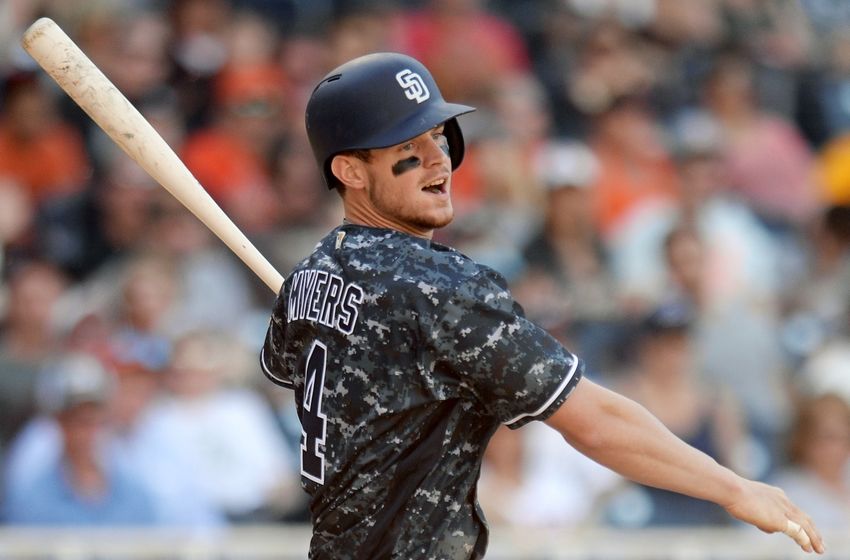This close-up photograph captures a baseball player from the San Diego Padres during a game, clad in a distinctive dark camouflage uniform. The back of his jersey prominently displays the name "Myers" and the number four. He has black tar beneath his eyes to shield them from the sun and is wearing a batting helmet for protection. His dark hair is neatly trimmed, accompanied by a short mustache and beard. The player appears to be in the midst of action, with his right arm extended forward, possibly having just hit the ball. The bat in his hands shows signs of wear, marked by numerous black streaks near the end. The background features a blurred crowd of spectators, who are out of focus and muted, accentuating the sharp and vivid details of the player in the foreground. He has a look of satisfaction on his face, his mouth slightly open as he gazes into the distance.